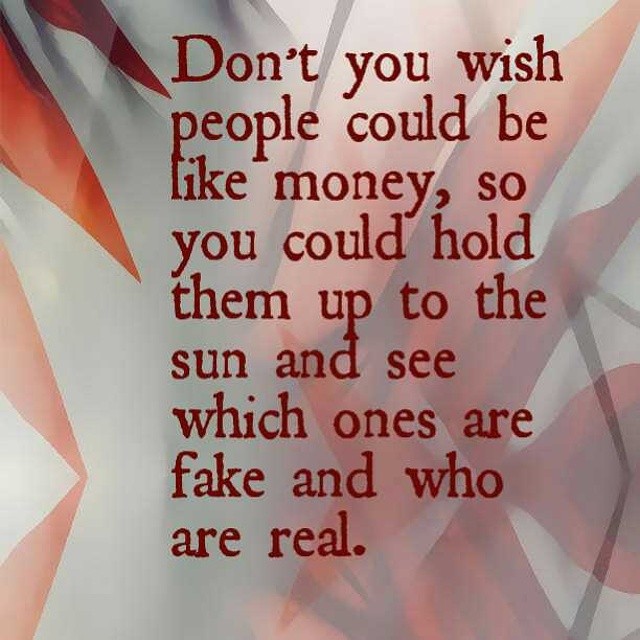The image features an abstract background composed of a combination of white, red, and grey colors, with triangle shapes creating a refracting effect that gives off the semblance of a gradient glow radiating from a light source at the top. Overlapping this background is a grainy texture that adds a unique visual quality. At the center of the image, there is a quote written in dark red text, where the first letter is capitalized and the remaining letters are in lowercase. The text reads: "Don't you wish people could be like money so you could hold them up to the sun and see which ones are fake and who are real." This graphic, with its profound quote and eye-catching design, is reminiscent of the kind of content often shared on social media platforms like Facebook or Instagram.